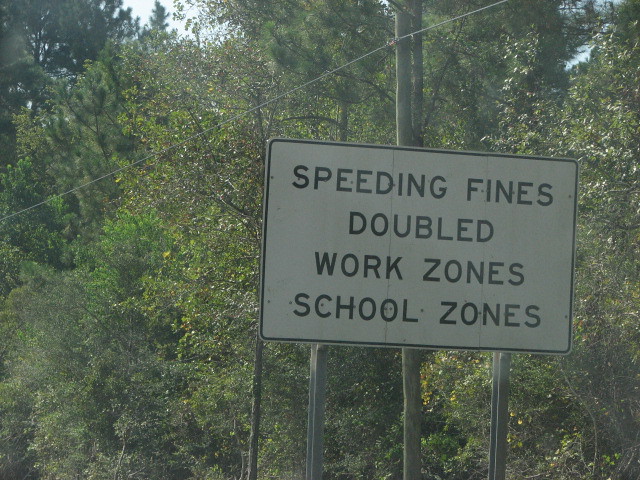In this horizontally oriented daytime photograph, we are looking into a dense area of mixed woodland featuring a variety of lush green pine and leafy trees, suggesting a spring or summer setting. The scene is predominantly composed of trees with their foliage fully in bloom, and patches of clear blue sky are visible towards the upper left corner, adding a touch of brightness to the image. Slight clouds can be observed, but the overall ambiance is sunny. Central to the image, slightly off to the right, stands a large white rectangular metal sign with a black outline and bold, uppercase black text. The sign, supported by two gray metal posts, reads: "SPEEDING FINES DOUBLED WORK ZONES SCHOOL ZONES." Behind this sign, a tall wooden utility pole stretches up through the center of the image, with silver cables running diagonally from the lower left to the upper right, likely for telephone or electrical lines. This picturesque scene, possibly captured from a moving vehicle or by someone walking along the street, suggests a residential or semi-rural area with a focus on road safety signages amid the natural wooded backdrop.